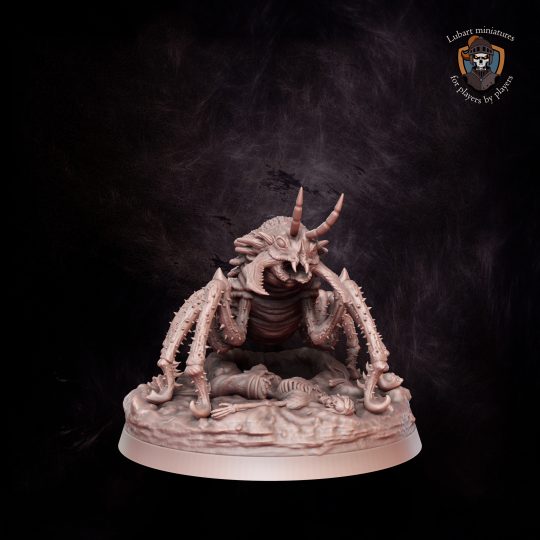The image showcases a detailed miniature, likely intended for use in tabletop gaming, depicting a terrifying, demonic, and insect-like creature. The creature towers at three times the width of a human, with six hairy, thorn-covered, spider-like legs ending in hook-shaped feet, all made from organic material. Its face, which points directly at the camera, features large mandibles with spikes, and an open mouth filled with intimidating talons. The head is crowned with imposing demon-like horns. The creature stands menacingly over the skeletal remains of a human, suggesting it has just devoured its prey. This gruesome scene is set against a completely black backdrop, with subtle white etchings resembling smoke or scratches adding to the eerie atmosphere. The miniature stands on a circular base that appears almost ghostly or demonic. In the upper right corner, white text reads "Lubert Miniatures for Players by Players," accompanied by a shield emblem featuring a skeleton in armor.